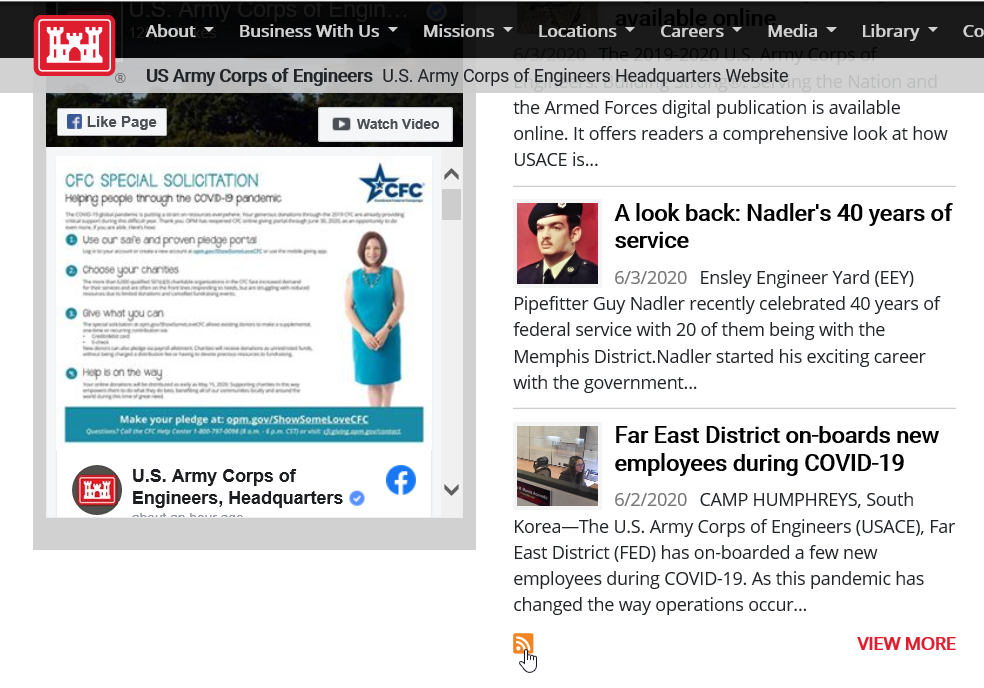This image captures the US Army Corps of Engineers headquarters website. The website has a crowded and somewhat dated design. The top left corner features a red rectangle with a white castle silhouette, serving as the site's logo. The main navigation menu includes sections such as "About," "Business With Us," "Missions," "Locations," "Careers," "Media," and "Library." 

On the left side, there is a social media integration panel displaying activity, including a partially visible Facebook post. A photograph of a woman is prominently featured, giving the impression that she is explaining the website's content. However, much of the text across the site is too small to read clearly.

The right side of the webpage lists articles, including highlights such as a post about "Inslee Engineer Yard Pipe Fitter Guy Nadler," who celebrated 40 years of federal service in June 2020, and another about the "Far East District onboarding new employees during COVID," also from June 2020. The mix of large and small text elements, along with the overall layout, gives the site a dense and somewhat cluttered appearance.